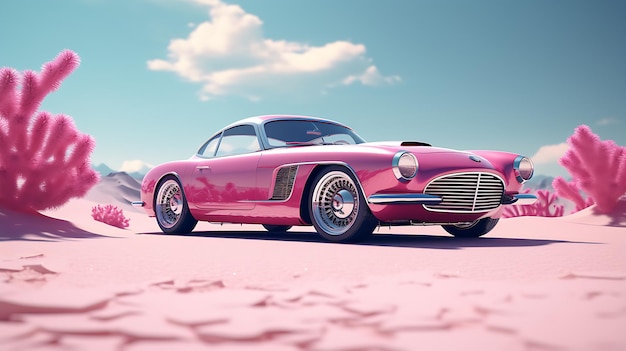In this digital painting, a bright pink, vintage-style sports car, resembling a classic Thunderbird or a Barbie car, sits prominently on a pink sand beach under a vivid blue sky with a singular puffy white cloud. The car is a vivid pink two-seater coupe with a white convertible top and chrome detailing, including round headlights encased in chrome rings, a shiny silver oval grille with horizontal and vertical lines, and chrome-colored spoke rims. The body of the car possesses rounded curves and a distinct hood scoop. Surrounding the car, pink cactuses and tall pink pampas grass grow out of the pink sand, adding to the otherworldly, surreal setting. The professional-quality image reflects the surrounding pink flora on the car's glossy surface, emphasizing its dreamlike, Photoshop-enhanced nature.